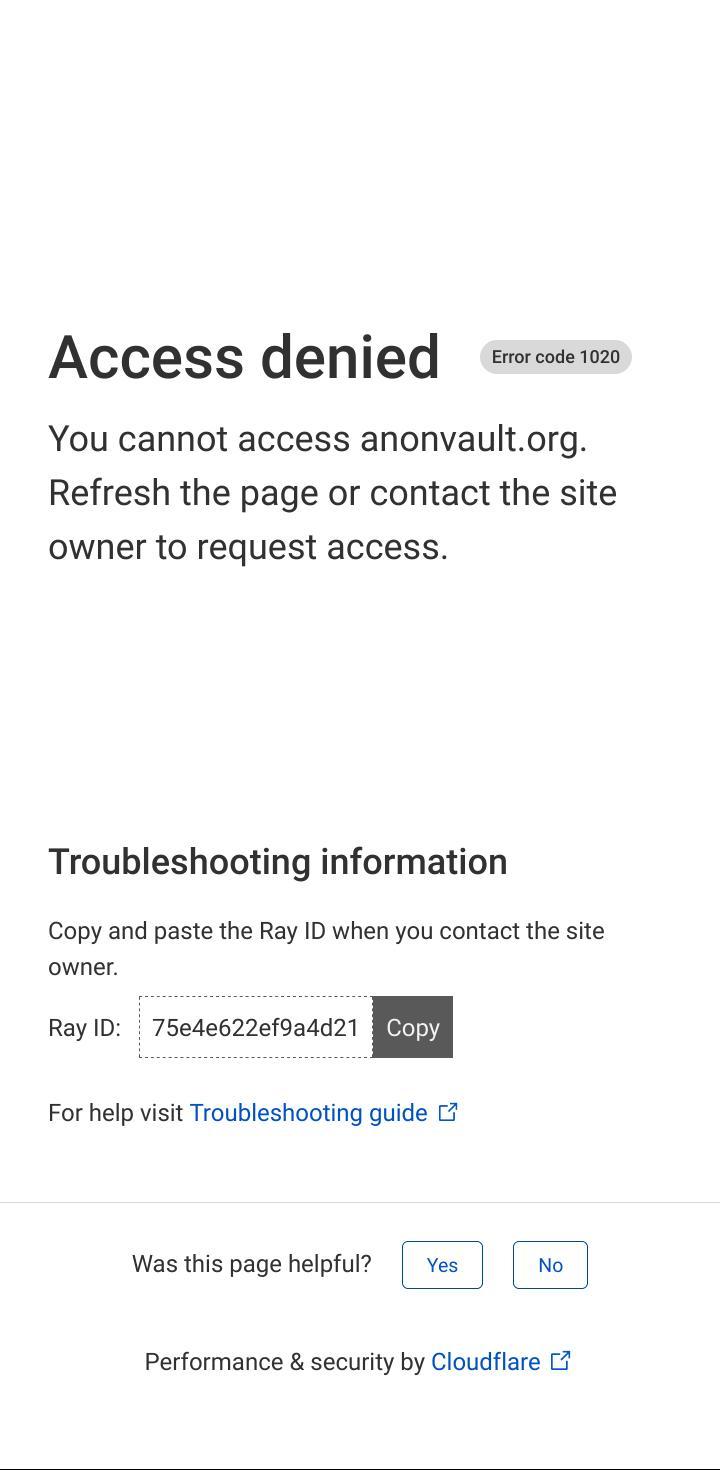The image appears to be a screenshot of an error page from Enonvault.org. In the top-left corner, there is a message reading "Access Denied" in black text, indicating an error has occurred. Adjacent to this, on the top-right, the phrase "Error Code: 1020" is displayed on a greyish-colored border. Beneath these messages, the text "You cannot access enonvault.org. Refresh the page or contact the site owner to request access." provides instructions for troubleshooting the issue.

The bottom half of the image contains further instructions under the heading "Troubleshooting Information." Here, it advises to copy and paste the RayID when contacting the site owner. The word "RayID:" is followed by a rectangular box containing a series of numbers on the left side, with the word "Copy" in white text on a dark grey background positioned within a small square on the right side of the rectangle.

Below this, a link styled in light blue text reads "Visit troubleshooting guide" for additional help. Finally, at the very bottom, the page asks "Was this page helpful?" with two boxes marked "Yes" and "No" for user feedback.